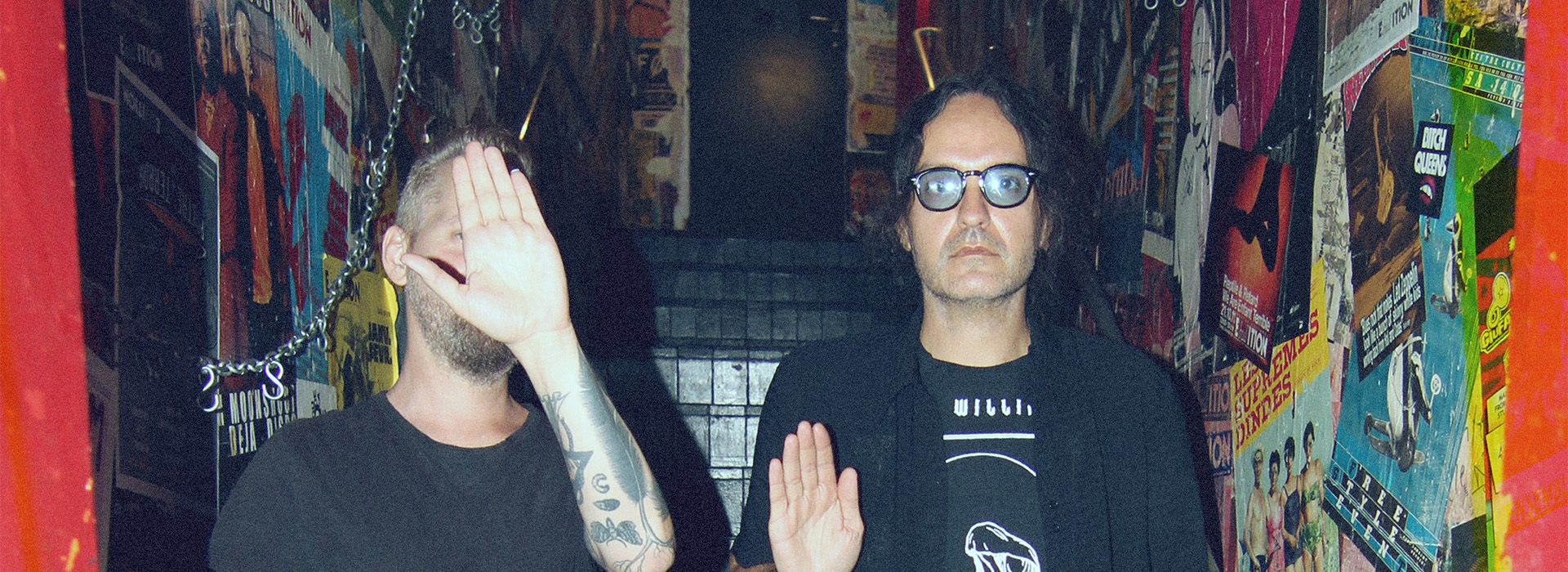In the image, two men, possibly rock stars, are seen on a staircase adorned with numerous old posters and stickers, evoking a concert venue or a bar atmosphere reminiscent of the Sunset Strip. The man on the left, in his mid-30s, has tattoos on his arm, including a feather, and obscures his face with his hand. He wears a plain black T-shirt. The man on the right sports large, Ray-Ban styled glasses, a faded mustache, black hair, a black blazer, and a black T-shirt featuring the name "Willy," potentially in reference to Willie Nelson. Both men's expressions suggest they were caught off guard, possibly by a camera flash, creating a spontaneous and candid moment. A red doorway and stair railings complete the scene, adding to the venue's gritty charm.